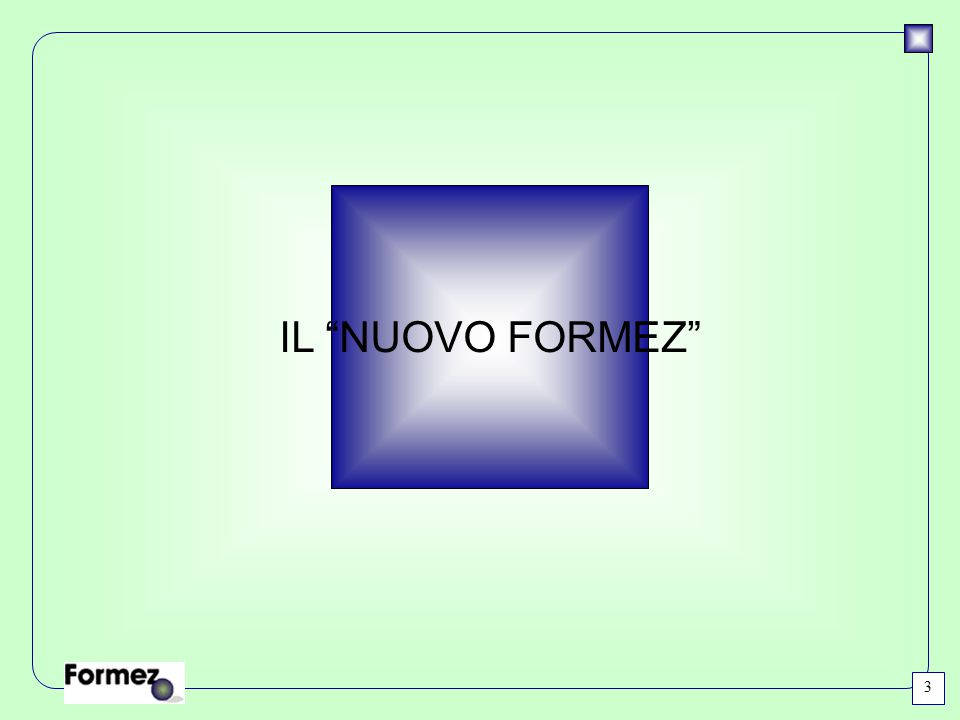The image features a large, light green rectangular background, which appears to be a slide for a presentation or demonstration. This background is bordered by a thin line. Centrally positioned within the slide is a blue square with a gradient, transitioning from blue at the edges to white at the center, forming an X-like pattern with two intersecting lines at a 45-degree angle. Superimposed on this blue square is the text "Il Nuovo Formez" in black font, with "Nuovo Formez" enclosed in quotation marks.

In the upper right corner of the slide, there is a smaller version of the same blue square with the gradient X. The bottom right corner of the slide displays a white box containing the number three. The bottom left corner features the word "Formez" spelled out in a white logo with blue gradient coloring. Adjacent to the letter 'Z' in "Formez," there is a blue sphere, adding a three-dimensional effect to the logo, possibly indicative of a trademark symbol.